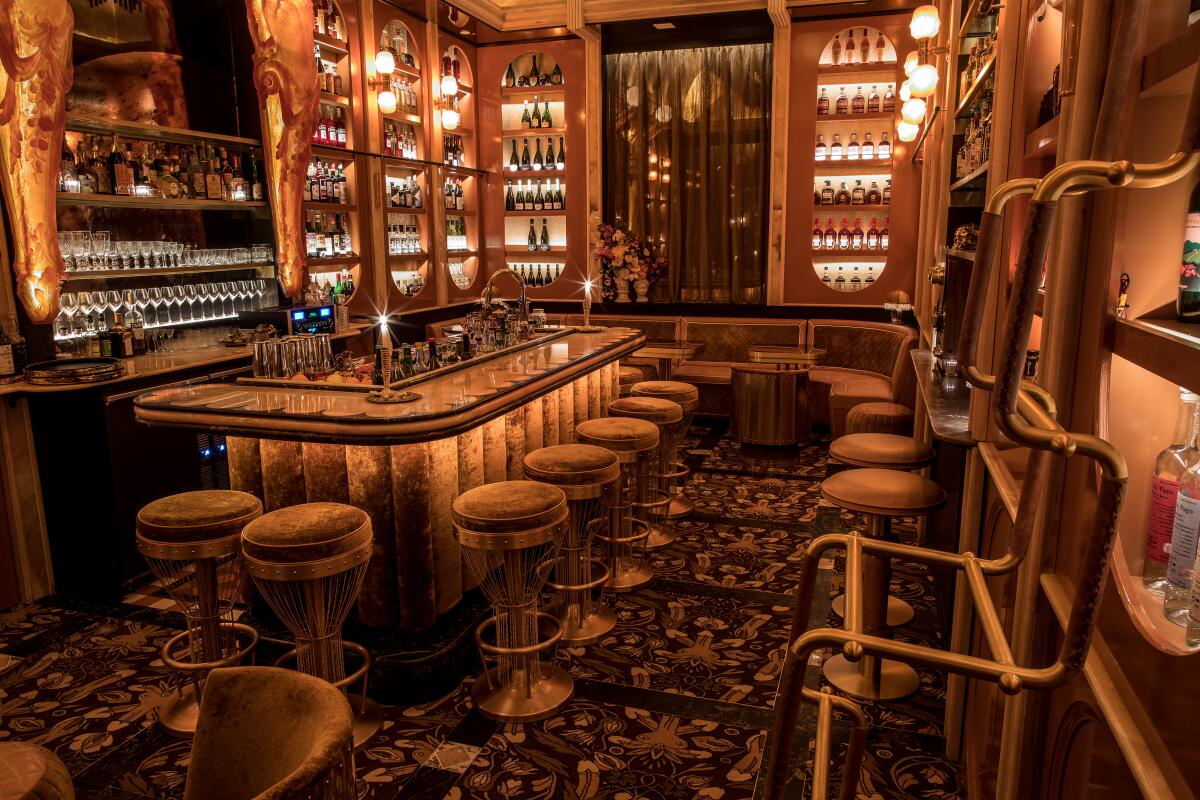The sepia-toned image depicts the luxurious interior of an elegant and exclusive bar, possibly located within a high-end club or casino. Dominated by a rich brown color palette with accents of bronze, copper, and gold, the bar area showcases a variety of detailed and stylish features. The bar counter, positioned centrally, is surrounded by round bar stools with cushions of golden velvet, supported by studded metal bands and footrests. The mirrored back of the bar shelves many different types of bottles and pristine glasses, vividly reflecting soft gold lighting from discreet downlights.

The plush carpet, featuring an intricate geometric pattern in bronze and brown, adds to the opulent atmosphere. An oriental-style rug with multiple patterned segments enhances the classic feel. Surrounding the bar are various seating options, including curved and straight benches with darker brown cushions on the backrests and lighter brown cushions on the seats, creating comfortable spaces for patrons. A copper metal tubing structure is noticeable in the right corner of the image, adding to the metallic visual appeal.

The walls, adorned with sheer brown curtains, shelves of bottles, and softly glowing lamps, complete the sophisticated decor. Additional details include candles on the bar, flowers next to a window, and a serene ambiance suggesting this space caters to an elite clientele seeking a refined drinking experience.